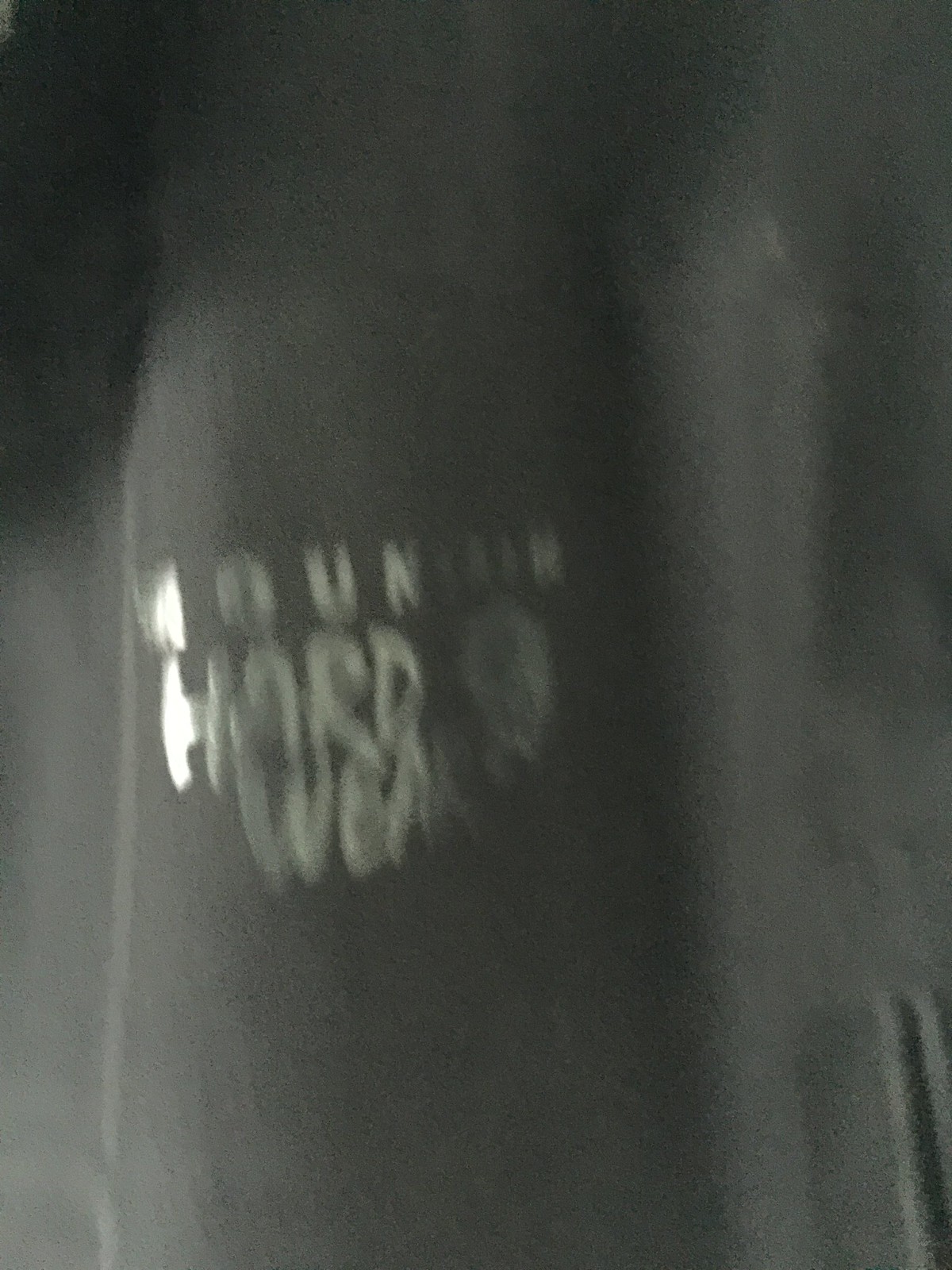This tall, vertical image portrays a dimly lit scene with a primarily black background, creating a moody, almost mysterious atmosphere. Dominating the center of the photograph is a blurry object, predominantly shaded in black and gray with shadows adding depth and texture. The central figure appears to be fabric with subtle curves, and the edges are softened, perhaps due to motion or low light.

Intriguingly, there is gold lamé appliqué lettering arranged in a circular manner on the left side of the fabric, contributing a touch of brightness and contrast against the darker tones. Although the blurriness impedes clear legibility, the partial visibility reveals the top word might contain an "O," "U," "N," suggesting it is approximately seven letters in length. The word below clearly seems to start with "H-A-R-D" embodying a sense of firmness or emphasis. Below, the letters seem to spell out "WORK," with the initial "W" and the rest of the letters slightly distorted but recognizable as "E," "R," and "K," followed by indistinguishable characters.

To the right, faint traces of additional gold lettering appear but remain too obscured by the blur to identify. The combined effect of the dark backdrop, blurry, curved fabric, and shimmering gold letters creates an enigmatic and evocative image, challenging the viewer to engage with its obscured details and form.